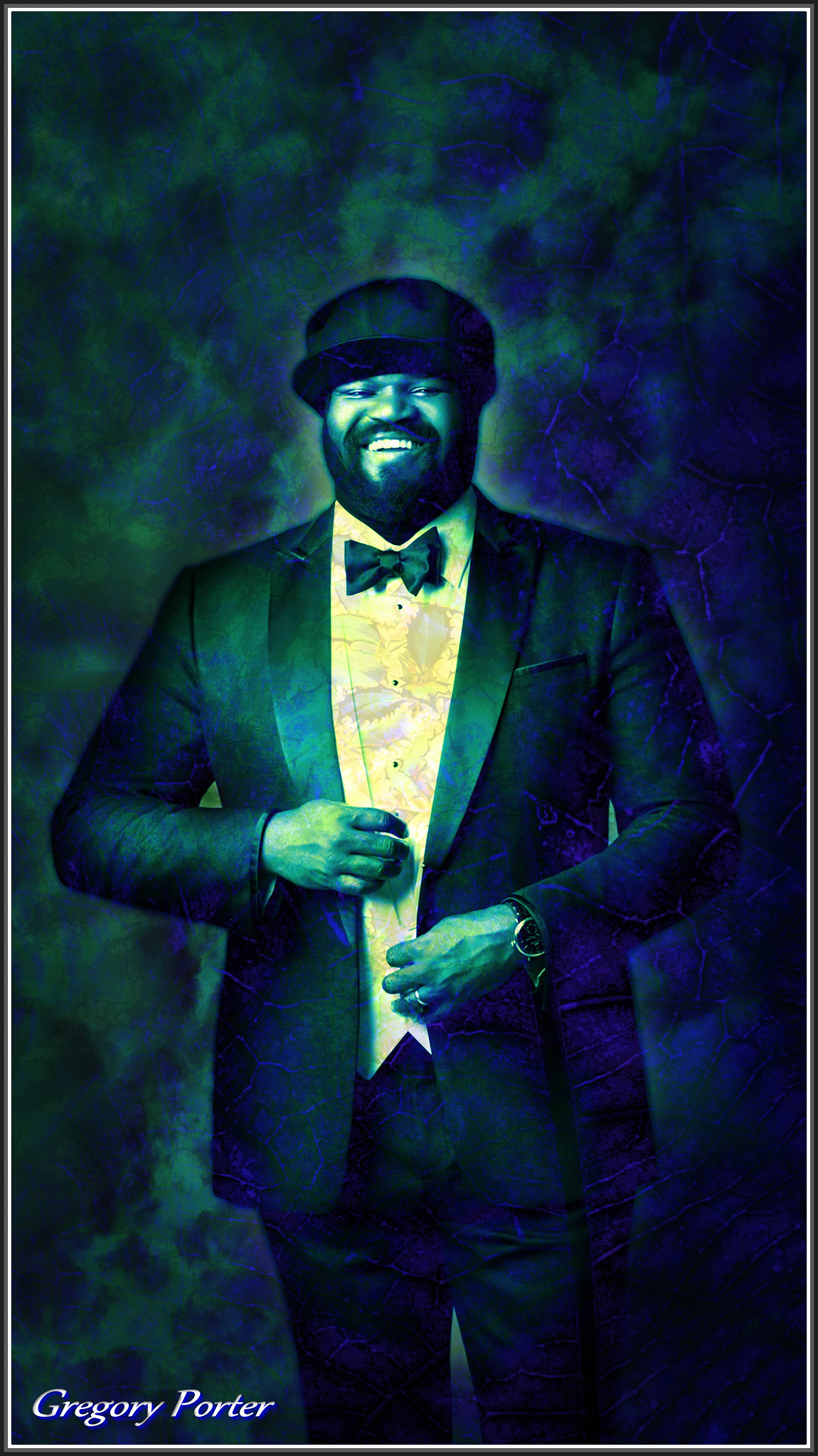The image displays a highly detailed, digitally generated or meticulously painted portrait of Gregory Porter, an African-American man. The background is composed of an intricate mixture of greenish and bluish hues, with textured patterns reminiscent of crumpled paper. At the center, Gregory Porter stands, captured with photorealistic precision. He is dressed in a formal black tuxedo, paired with a black bow tie, a white dress shirt, and a white waistcoat. He accessorizes with a black cap that is more stylish than a typical baseball hat, a wristwatch on his left hand, and a ring on his ring finger. Porter is depicted smiling as he looks to the side, holding the buttons of his waistcoat with both hands. His name, "Gregory Porter," is inscribed in the bottom left corner of the image.